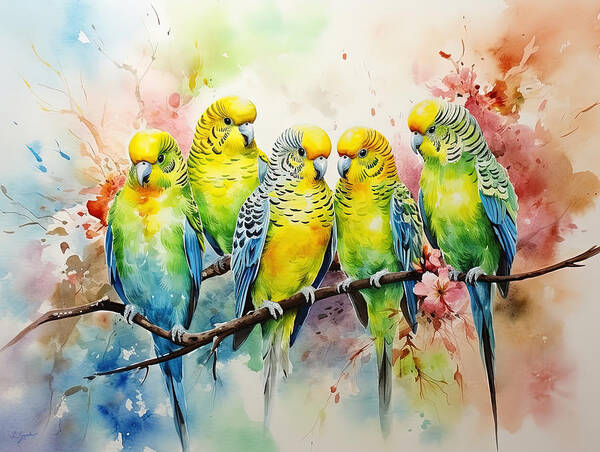This image is a digital screenshot of a watercolor painting featuring five intricately detailed parakeets perched on a single brown branch. Each parakeet sports a vibrant combination of colors with yellow heads and a mix of yellow, green, and blue on their bodies. Their wingtips exhibit shades of blue and gray, and some birds have distinctive white markings around their necks. The background is a highly abstract, tie-dye-like composition with splatters of pink, green, blue, and hints of white, creating an ethereal backdrop that highlights the clarity and detailed texture of the birds' feathers. Their small, delicate feet are clearly visible gripping the branch, adding to the overall lifelike quality of the artwork.